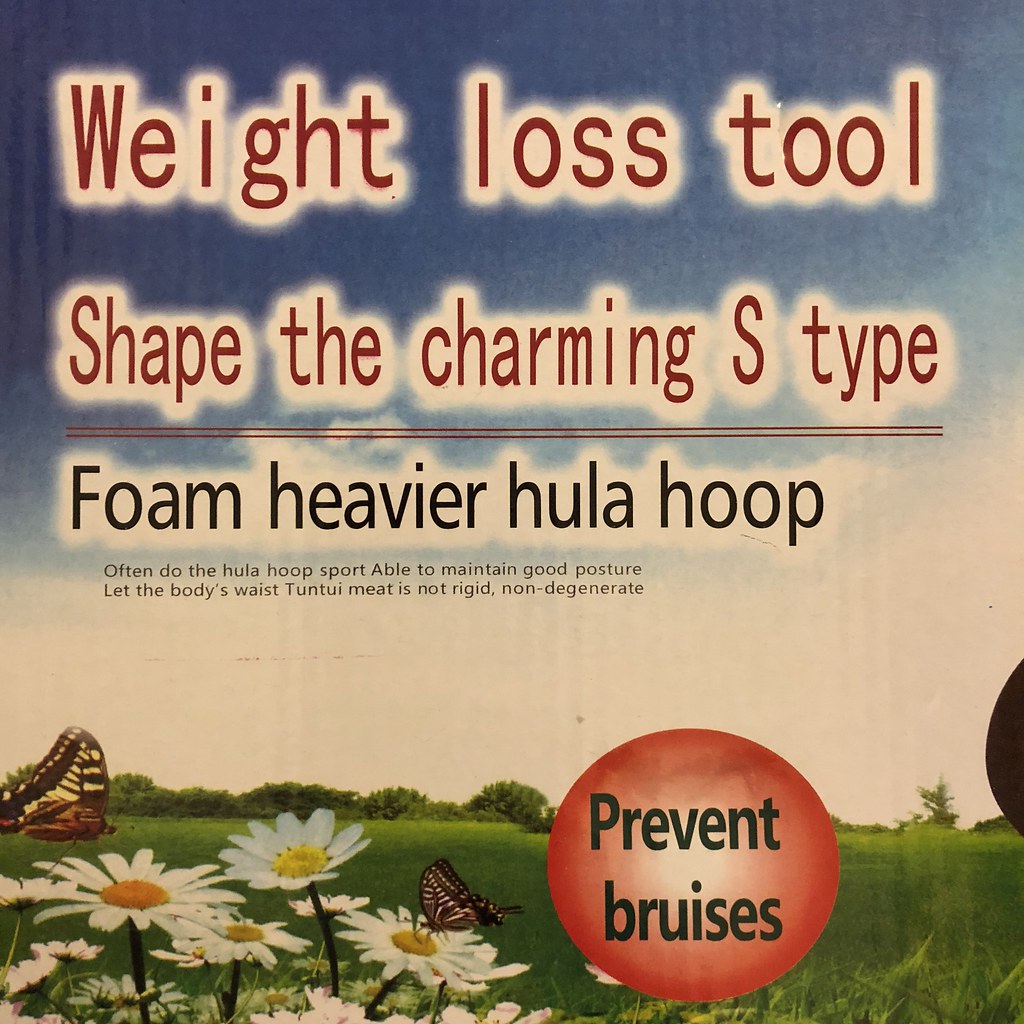The image is an advertisement with a vintage feel, promoting a weight loss tool. Dominating the upper portion, bold red text reads: "Weight Loss Tool, Shape the Charming S-Type," set against a white backdrop. Below this, in black text, it describes a "foam, heavier hula hoop" which is designed to help maintain good posture and prevent the body's waist from becoming rigid or degenerative. Further down, a red circle with the words "Prevent Bruises" encases black text.

The lower section of the image features an idyllic natural scene: a blue sky, lush grass, and scattered trees. Sunflowers bloom vibrantly, attracting two butterflies with brown and black wings. The overall aesthetic is completed with a round cut-out shape on the right side, adding a unique touch to the vintage design.